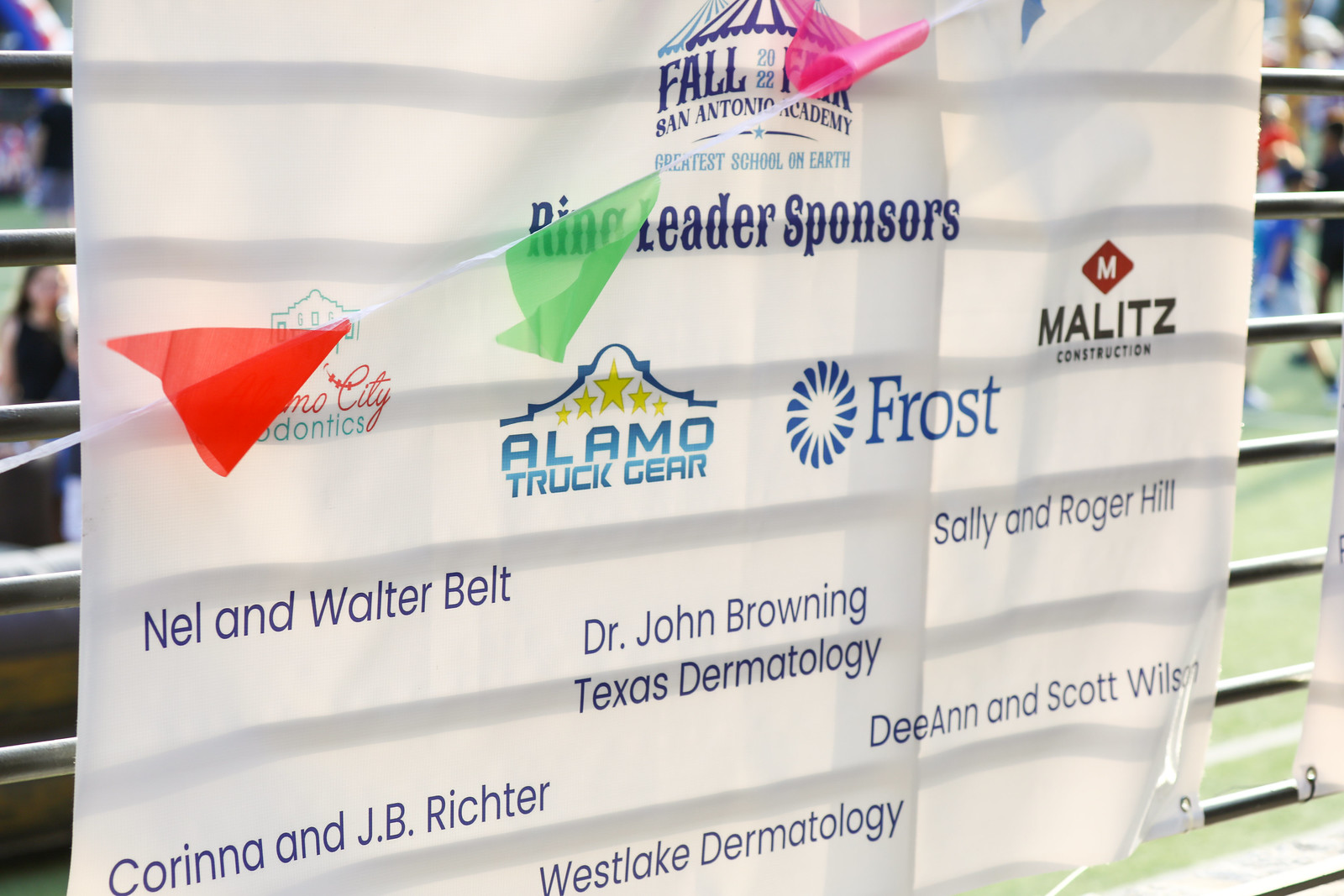The image features a large white banner attached to a gray metal fence, typically seen at events like a rodeo or school fair. The banner serves as a sponsor display for the "Fall 2022 Fair at San Antonio Academy," prominently titled with "Ringleader Sponsors" beneath it. The background reveals a green grassy area with blurry figures and additional banners.

The top of the banner showcases a tent-like cover design above the fair's name. Streamers with red, green, and pink flags are draped across the middle left to the top center of the banner, partially covering some of the text and logos.

The sponsors listed on the banner include:
- **Alamo Truck Gear**
- **Frost** (possibly Frost Bank)
- **Militz Construction**
- **Sally and Roger Hill**
- **Dr. John Browning, Texas Dermatology**
- **Karina and J.B. Richer**
- **Westlake Dermatology**
- **Deanne and Scott Wilson**
- **Nell and Waterbelt**

Despite some parts being obscured by colorful streamers, the banner remains a clear display of community support for the fair, organized by the San Antonio Academy.